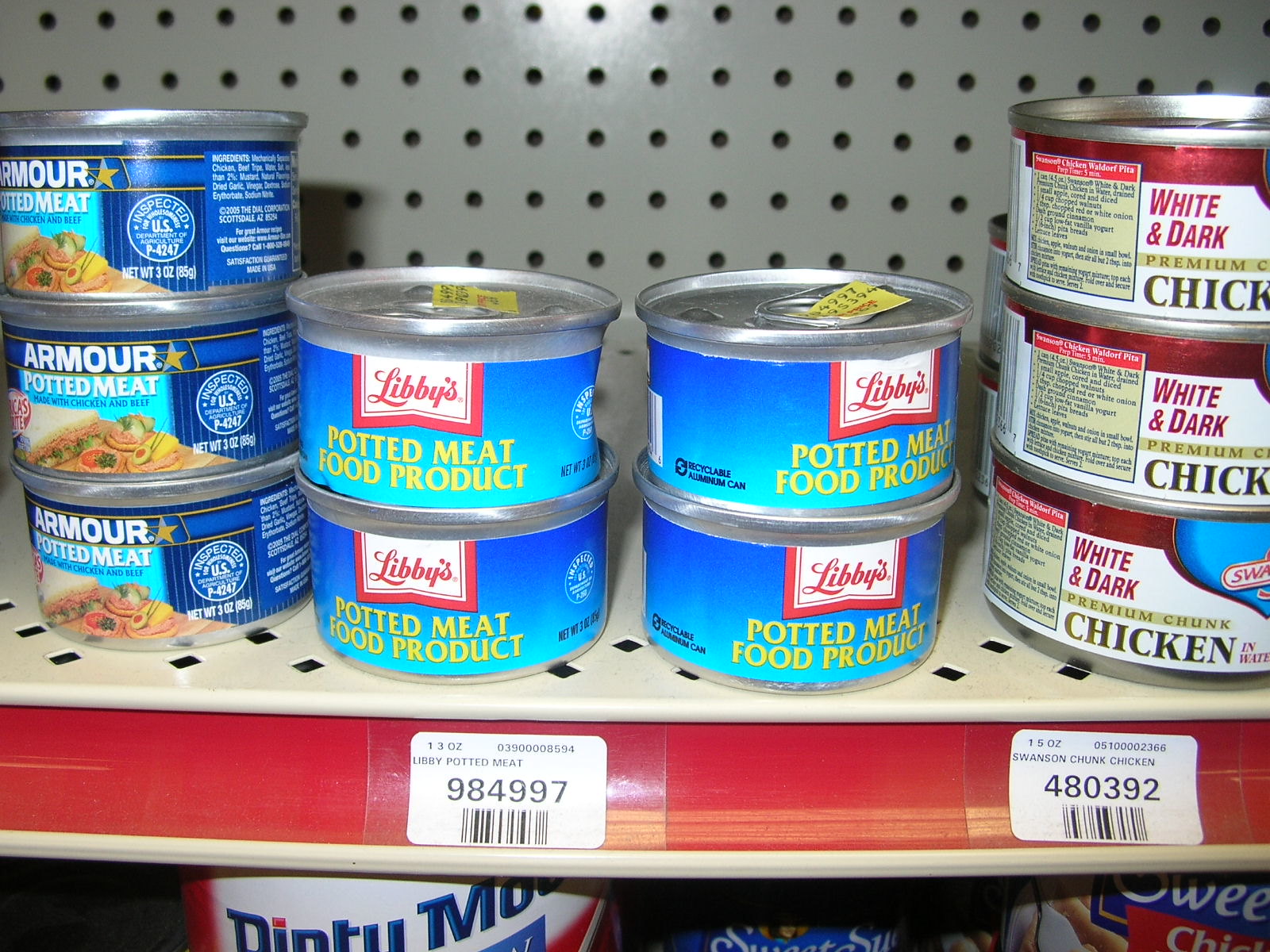On a beige metal shelf with a distinct red strip running along its front edge, there's an organized variety of canned goods. The shelf holds three cans of Armor potted meat, neatly arranged. Adjacent to these, there are four cans of Libby potted meat, stacked in two neat columns of two cans each. Nearby, three cans of Swanson's white and dark premium chunk chicken are carefully placed. Positioned underneath these items is a solo can of Dinty Moore Beef Stew. Additionally, there are cans of Sweet Sue and Sweet Sue Chicken, adding diversity to the assortment. The shelf features a red tag with a white barcode prominently displayed in front, listing product codes for easy identification: potted meat is labeled as 984997, and Swanson's chunk chicken as 480392.